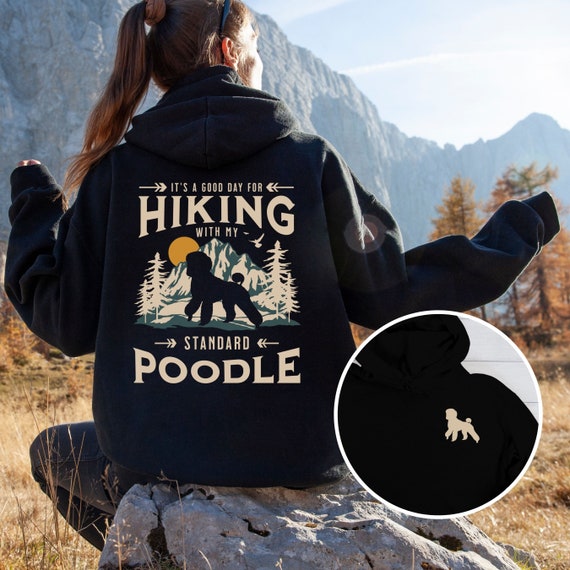In this captivating image, likely intended as an advertisement, the focus is on a serene natural setting featuring a girl perched on a rock amidst a landscape of dried-out grass and autumnal brown trees, creating a warm yet desolate atmosphere. A majestic mountain range looms in the background, its rugged rock formations reaching towards the clear blue sky dotted with fluffy white clouds. The main highlight is the girl's attire: a black hooded sweatshirt, seen from behind, with her long brown hair cascading down. The hoodie bears the printed phrase, "It's a good day for hiking with my standard poodle," accompanied by a silhouette of a black dog standing in front of a mountain, mirroring her own stance. Additionally, an inset circle to the right displays the hoodie’s front, showcasing a silhouette of a white dog. This detailed image not only captures the essence of an adventurous spirit intertwined with nature but also emphasizes the appeal of the outdoor-themed apparel.